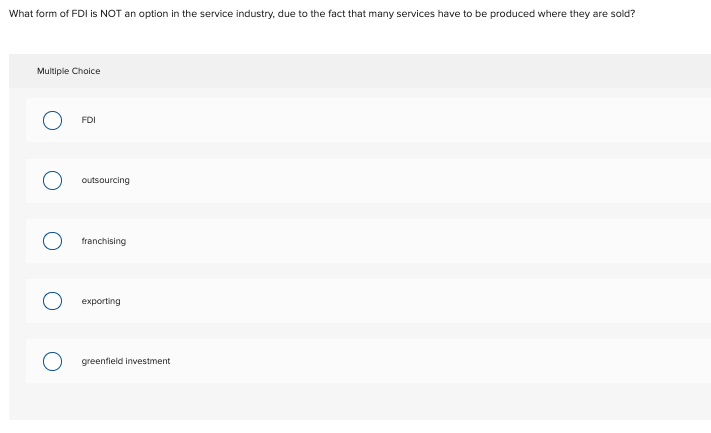A screenshot captures a multiple choice question from an electronic quiz focused on Foreign Direct Investment (FDI) in the service industry. The question, displayed in black font within a white bar at the top of the page, reads: "What form of FDI is not an option in the service industry due to the fact that many services have to be produced where they are sold?" Below the question, five options—FDI, outsourcing, franchising, exporting, and greenfield investment—are each enclosed in rectangular boxes with empty circles beside them, awaiting user selection. The interface is minimalist, featuring a simple white background with no additional images or decorative elements.